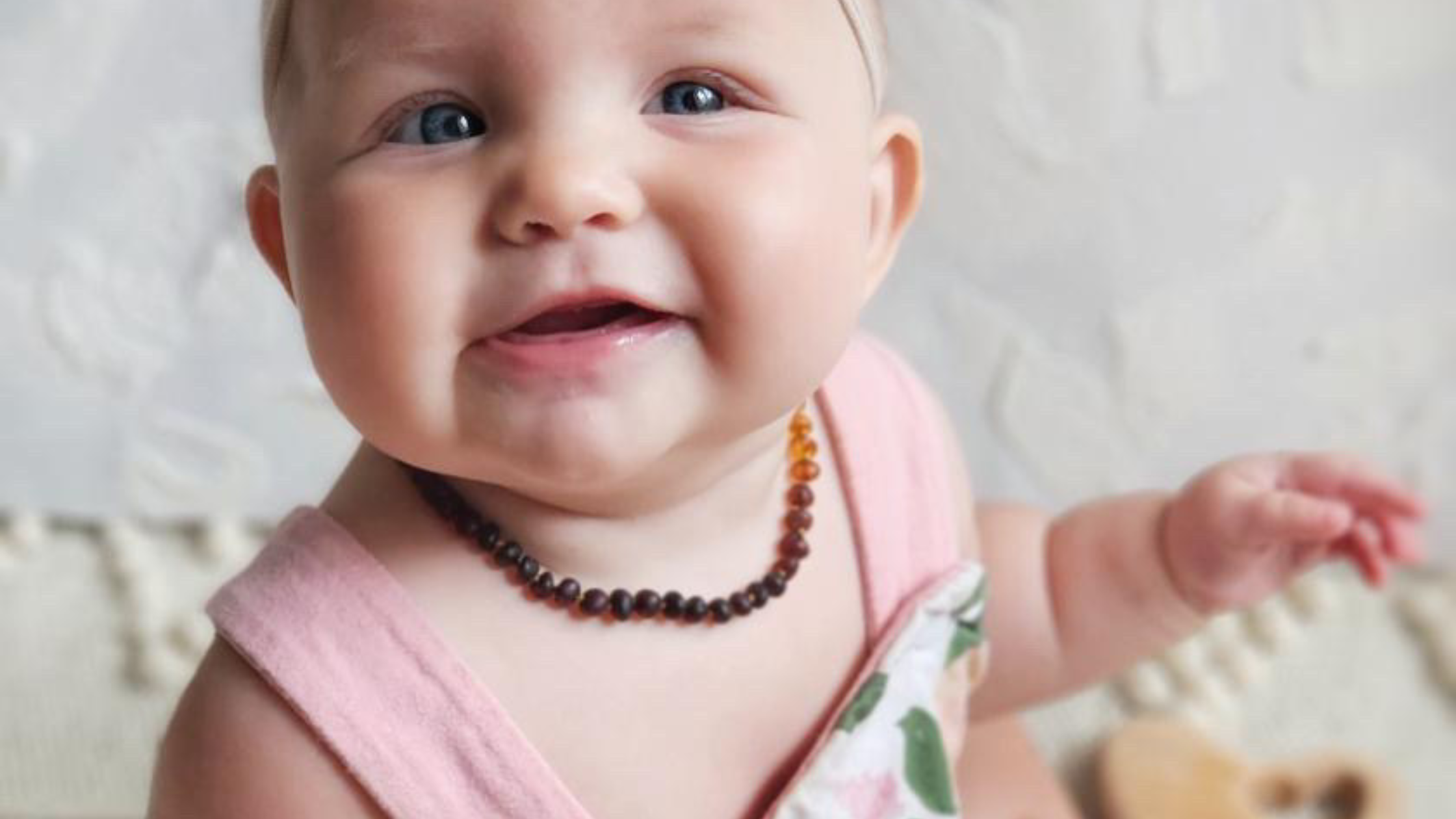In this realistic and detailed photograph, a baby girl is the central focus. She is seated in the middle of the frame, her light skin contrasting with the muted backdrop. Behind her, a white wall adorned with subtle, white-on-white designs creates a textured background, blending seamlessly into the scene. To her rear, a single shoe—presumably hers—is just visible. The baby girl, with her chubby cheeks and slightly gaping mouth, showcases an endearing expression. Her very blue eyes are bright and inquisitive, peering out from beneath short, wispy blonde hair. She is adorned with a brown and black beaded necklace, adding a pop of color against her pink overalls. The overalls themselves are embellished with charming pink and green floral patterns. Her left hand is raised, revealing adorably fat wrinkles on her arm, capturing the innocence and beauty of early childhood.